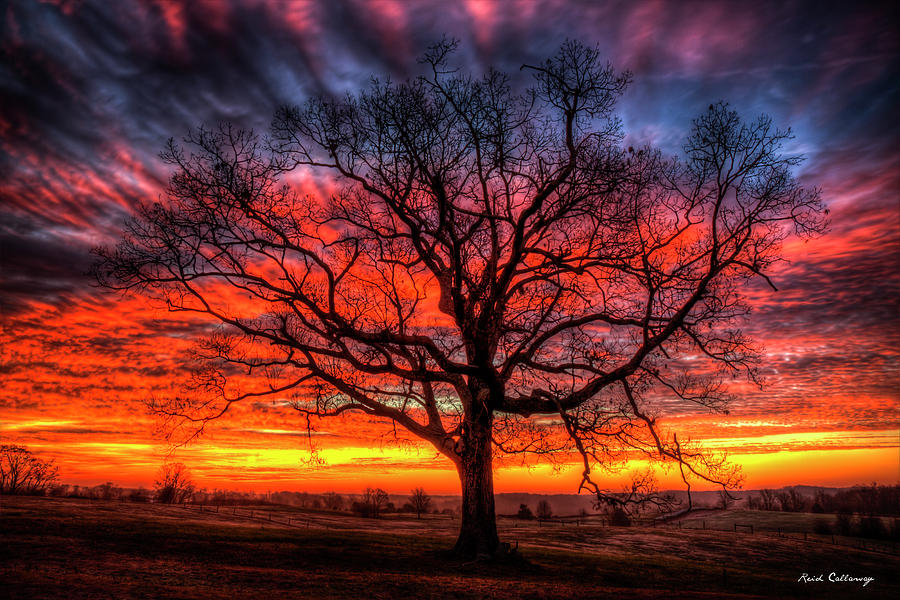This striking photograph captures a vibrant sunset scene over a flat prairie or rural farmland landscape. Dominating the image is a majestic, leafless tree positioned centrally, reaching impressively towards the sky with its intricate, gnarly branches. The tree’s silhouette against the colorful sky highlights its significant size and unique structure. The sky transitions through a breathtaking ombre effect, starting with deep purples and blues at the top, melding into rich reds and pinks, and finally glowing in vivid oranges and yellows near the horizon. The lower fifth of the image shows the dark, minimalistic foreground, featuring mostly grass with a few scattered bushes and smaller trees. The vivid colors and tie-dye cloud patterns suggest a long exposure time, enhancing the scene's beauty and creating a dreamlike quality. This photograph, credited to Reid Callaway as noted by the signature in the bottom right corner, vividly captures the serene yet dramatic beauty of nature.